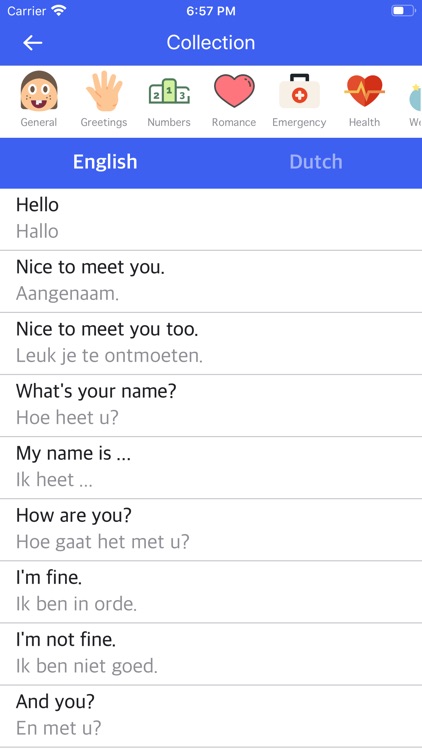The screenshot depicts a user interface of a translation application. At the top of the screen, the word "Collection" is prominently displayed, indicating a curated set of translation categories. Below this header, there are several icons representing different categories: General, Greetings, Numbers, Romance, Emergency, and Health.

The left side of the screen is labeled "English," while the right side is labeled "Dutch," indicating the languages involved in the translations. The English phrases are displayed in black text at the top of each translation pair, followed by their corresponding Dutch translations in grey text beneath them.

The phrases included in this particular view are as follows:
- "Hello"
- "Nice to meet you"
- "Nice to meet you too"
- "What's your name?"
- "My name is..."
- "How are you?"
- "I'm fine"
- "I'm not fine"
- "And you?"

These phrases span common greetings and introductory questions, providing essential conversational dialogue for users needing quick access to basic communication in Dutch.